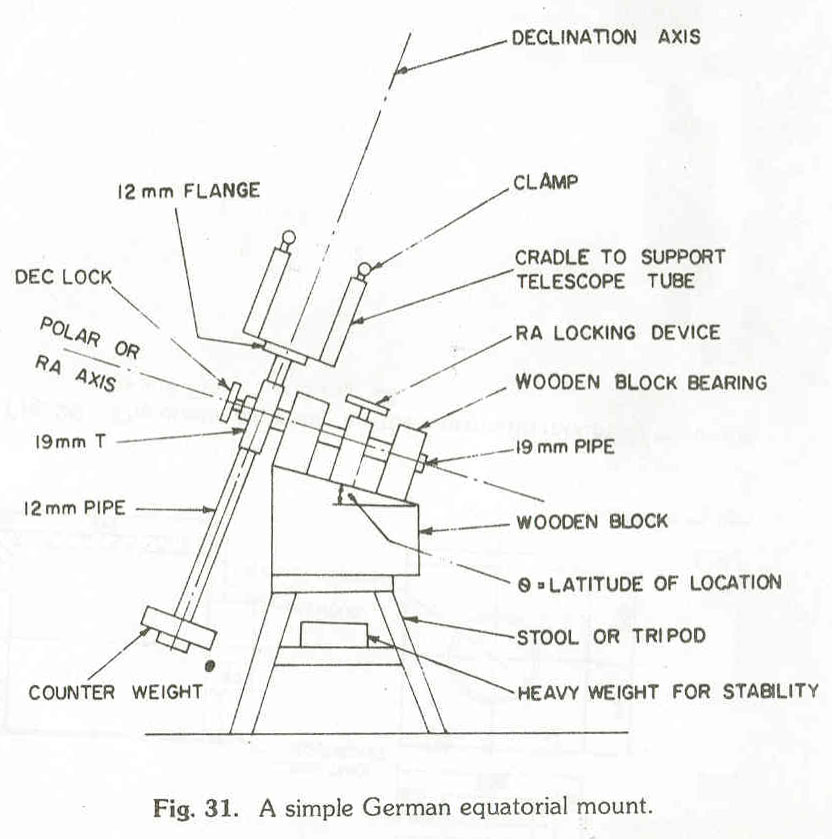This black-and-white engineering drawing, labeled "Figure 31," depicts a simple German equatorial mount for a telescope. The detailed mechanical illustration showcases a mount on a stool or tripod, with labeled components including a declination axis, RA (polar) axis, DEC lock, and numerous structural elements such as a 12mm flange and 19mm pipe. It features a heavy counterweight for stability, a cradle to support the telescope tube, and several locking devices. Annotations point to various parts like the clamp, wooden block bearing, and indicate zero as the latitude of location. The illustration combines technical precision with clarity, making all parts and their functions easily identifiable.